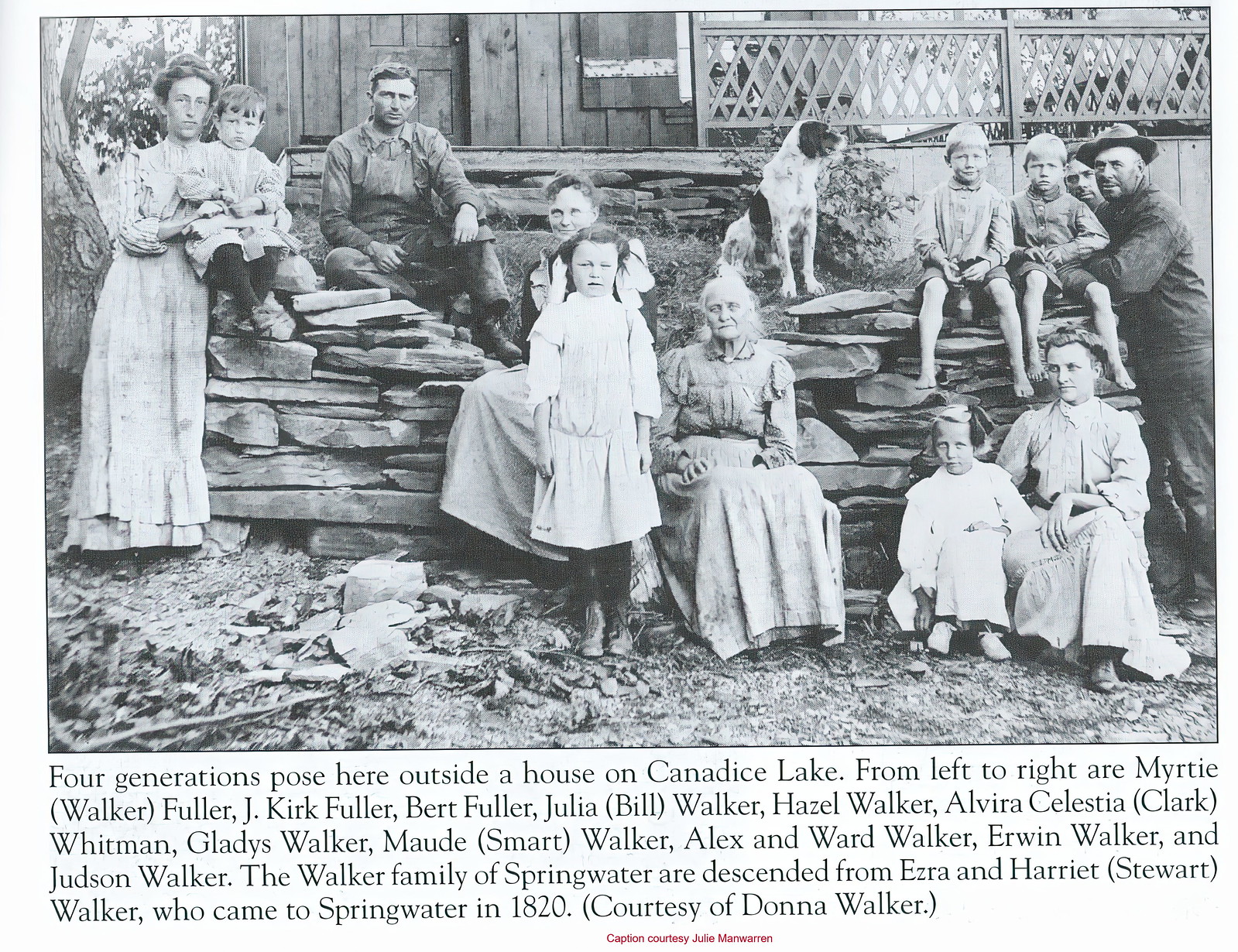This black-and-white photograph captures a nostalgic moment of a multi-generational family posing outside a house on the stone steps by Candace Lake. The image is rich with history, showcasing four generations of the Walker family from Springwater, descended from Ezra and Harriet Stewart Walker, who settled in Springwater in 1820. From left to right, the family members are Murty Walker Fuller, J. Kirk Fuller, Bert Fuller, Julia Bill Walker, Hazel Walker, Alvira Celestia Clark Whitman, Gladys Walker, Maude Smart Walker, Alex and Ward Walker, Erwin Walker, and Judson Walker. The scene includes a mix of very young children to elderly grandparents, all appearing content and interconnected. Captions, provided courtesy of Donna Walker and Julie Manna Warren, are inscribed below the image in a serif font, resembling Garamond, adding to the timeless quality of this cherished family portrait.